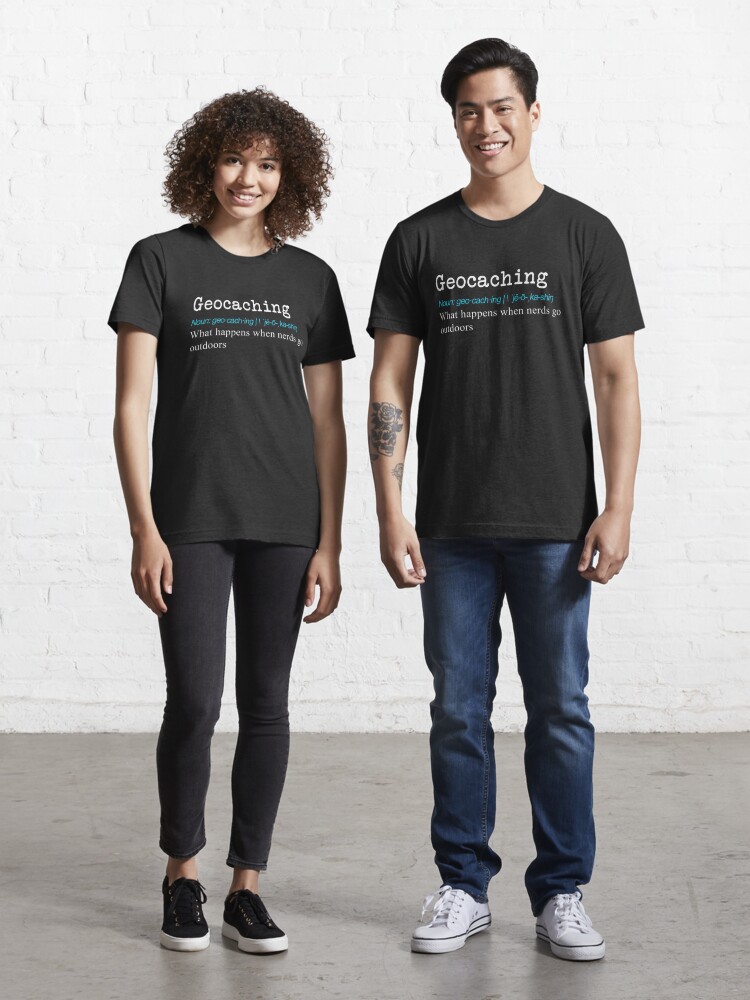In this detailed image, two individuals are standing side by side, posing with cheerful smiles against a white wall with gray cement flooring beneath them. On the left is a woman who appears to be of mixed-race or Hispanic descent, wearing black leggings, black sneakers with white soles, and a black T-shirt that says "Geocaching: what happens when nerds are outdoors." Her hair is really curly, ranging from brown to black. To her right stands a man of Asian descent, taller than the woman, wearing dark blue jeans and white sneakers. He is also wearing an identical black T-shirt with the same geocaching slogan. He sports a modern, short hairstyle and has a black-and-white rose tattoo on his right arm. Both individuals are posing confidently, likely as enthusiasts or advertisers of geocaching.